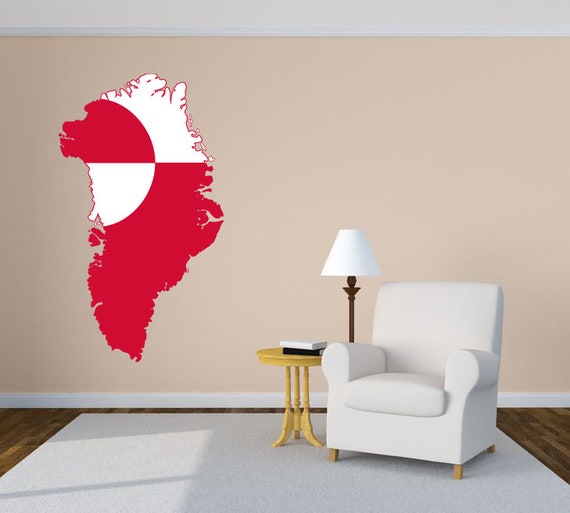This computer-generated image depicts a cozy corner of a room featuring light pink walls with white crown moldings at the top and bottom. The flooring consists of dark wood panels accompanied by a large, light gray rectangular rug. A plush, cushioned white chair with four wooden legs sits on the rug, next to a light wood round table with three legs. The table holds two books—a black one stacked beneath a white one. Behind the chair, there's a wood floor lamp with a slender brown metal post and a white lampshade. To the left side of the image, a red and white artistic depiction of Greenland adorns the wall, with the red occupying the lower half and a circle inverting the colors within the shape of the country.